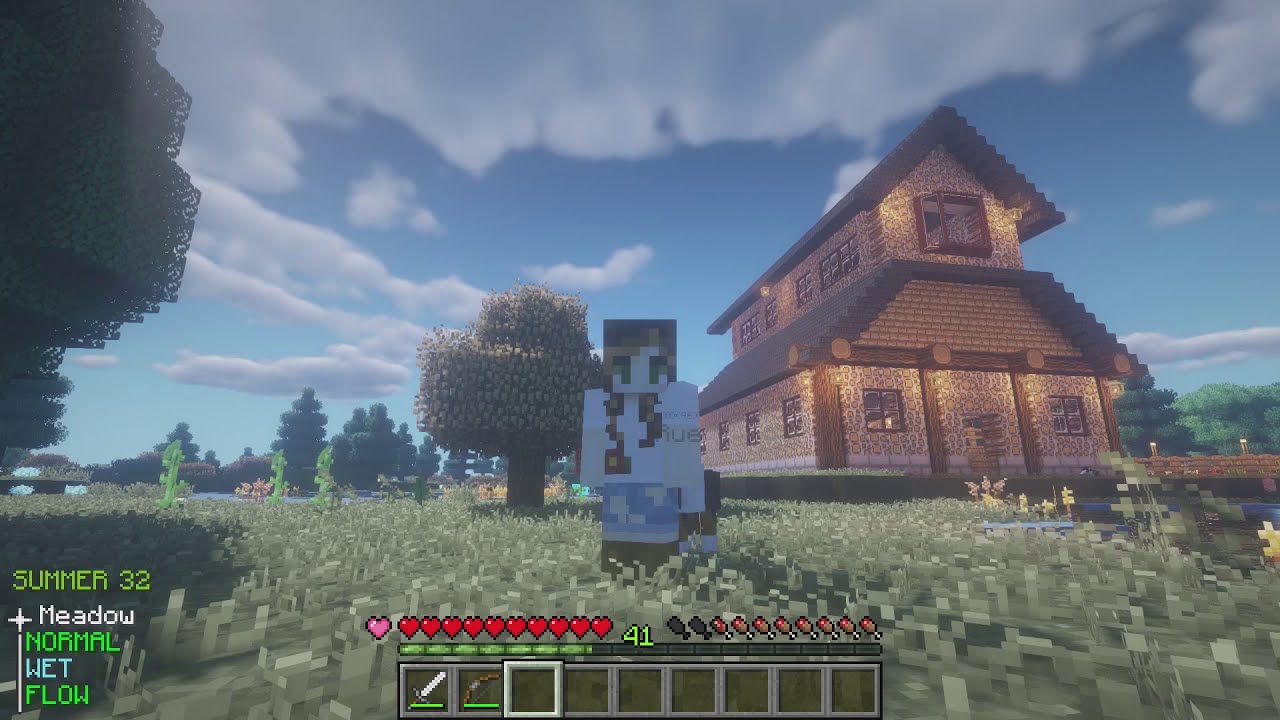In this highly detailed screenshot from the video game Minecraft, the central focus is on a character with green eyes and blonde pigtails, wearing a white shirt and blue jeans. The character, who has a blocky, Lego-like appearance, is standing in a grassy field facing the camera. To the right of the image, there is a wooden log cabin, which appears to be two to three stories tall. The cabin features a rectangular base, a parallelogram-shaped mid-section with slanted roofs on either side, topped by a smaller rectangular section with an A-shaped slanted roof. The roof of the cabin is black and is dotted with several points of light. In the background, there is a serene landscape featuring a blue sky with realistic clouds, verdant trees, water, and some tall, skinny light green plants. The bottom of the screen displays a user interface with weapon choices including a bow and a sword, some empty slots, a series of hearts likely indicating health, and what appear to be wine bottles, possibly for health or food. Additionally, the on-screen text reads "summer 32" in the lower left-hand corner followed by "meadow," "normal," "wet," and "flow," possibly indicating environmental conditions or game settings.